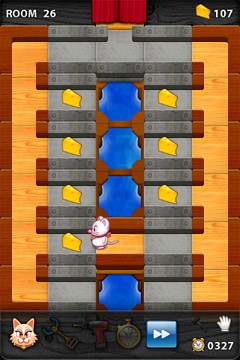The image is a screen capture from a mobile video game, displayed in portrait orientation. At the top of the screen, a black banner reads "room 26" on the left, and on the right, it shows an icon of a yellow cheese wedge with the number "107" next to it. The entire scene has a layered, wood-colored frame with brown outlines.

In the central part of the image, the overhead layout of a room is visible, filled with numerous mousetraps, each baited with a yellow cheese wedge. A white mouse with a red bandana and a small smile on its pink-nosed face is seen happily approaching one of the pieces of cheese amidst the traps. The background elements suggest either water or sky, with two vertical red lines resembling curtains marking some sort of division in the room.

At the bottom of the screen, there's a cartoon image of a cat's head with perked ears, pink inside the ears, and a collar around its neck. Nearby are various tools, including a drill, a grabbing claw, and a mallet. There's also a blue square containing a fast-forward icon (two arrows pointing to the right). To the right, a digital timer reads "0327," indicating the elapsed or remaining time.